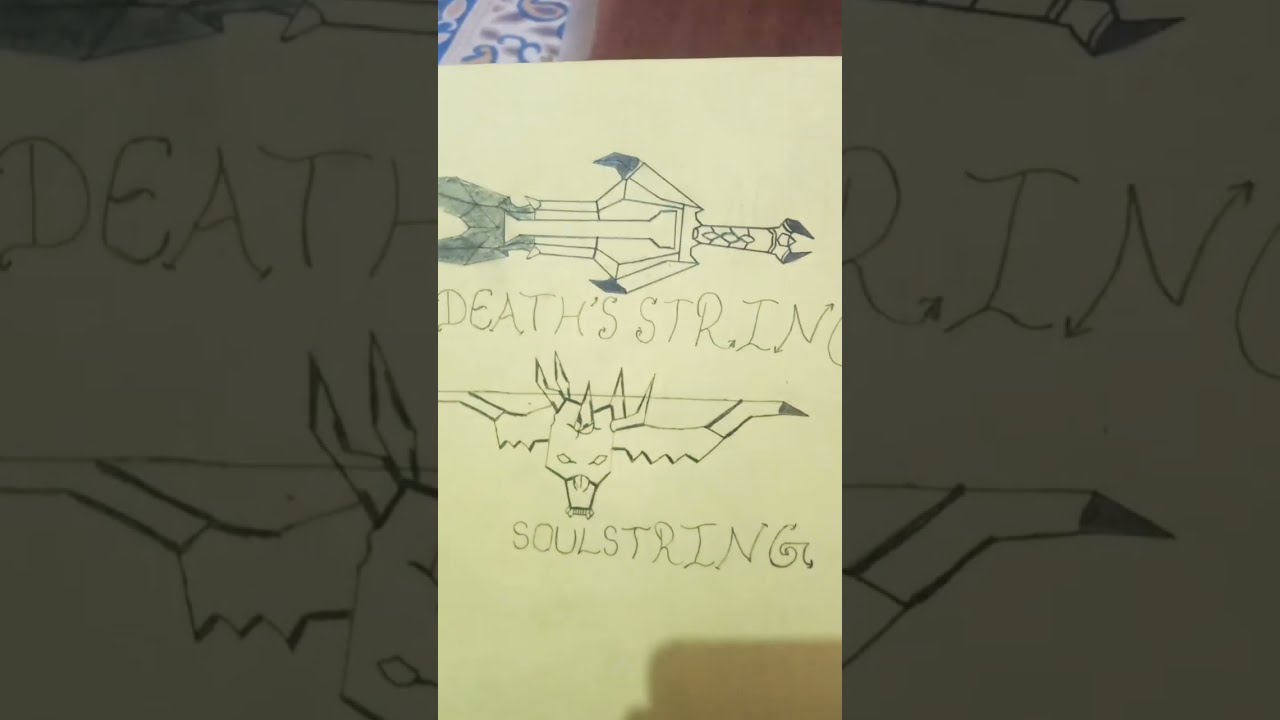The image predominantly displays a central photograph that appears to be a drawing on yellow paper, portraying two distinct fantasy weapons. The central third of the image houses the primary artwork, while the left and right thirds amplify this central area by showing zoomed-in and darkened versions of the same scene.

The top section of the drawing features a highly geometric, lead or graphite-rendered fantasy sword. The sword showcases a handle adorned with a claw-like design, extending into a guard with a similar claw motif. The blade itself bifurcates towards the end, creating a pointed, scissor-like pattern that is shaded darker. Beneath this elaborate sword is an ornate, stylized cartoony text that reads "Death's String."

Below the sword, there is an intricate drawing of a bow, which is depicted with a geometric design incorporating a face resembling a skull or bat. This face includes features such as horns, fangs, and menacing eyes, adding a dark, fantastical element to the weapon. The bow is strung with a string positioned on its top, and beneath it, in matching stylized text, is the inscription "Soul String."

The background of the image reveals a mix of brown and blue designs, suggesting the photograph was taken on a surface with these colors. There are different shades of gray across the drawing, emphasizing the contrast and details of the artwork. Overall, the photograph provides an intriguing glimpse into the imaginative world of fantasy weaponry, suggesting it might be a younger person's concept art, possibly captured from a mobile device.